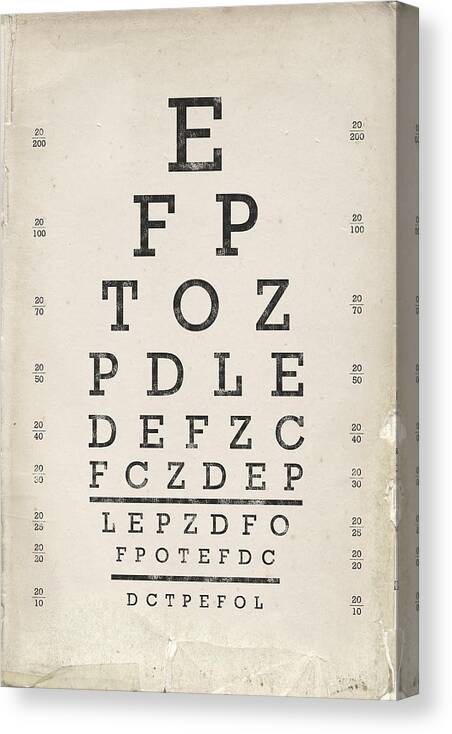This image depicts an aged and slightly tattered eye chart with a dulled, off-white background, likely hanging on a wall. At the top of the chart, prominently displayed, is the largest letter 'E', followed by progressively smaller rows of letters: FP, TOZ, PDLE, DEFC, FCZDEP, LEPZDFO, FPOTEFDC, and the smallest row being DCTPEFOL. Alongside these rows, from top to bottom, the numbers 20/200, 20/100, 20/70, 20/50, 20/40, 20/30, 20/25, 20/20, and 20/10 are indicated, denoting the visual acuity each row tests. The chart's appearance suggests it is old and well-used, possibly mounted in a picture frame and slightly angled to the left.